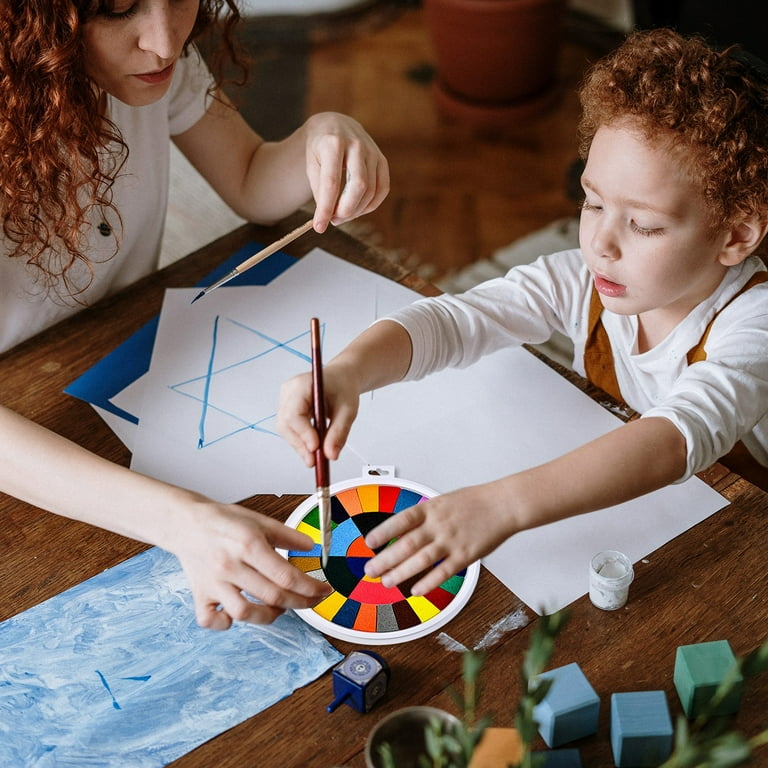In this image, a woman and a young boy, who both share light skin and strikingly similar curly red hair, are engaged in a painting activity at a brown table. The pair, possibly a mother and son, are both dressed in white shirts and appear to be enjoying their creative time together. On the table in front of them, the boy is enthusiastically painting on a white sheet of paper, with a Jewish six-pointed star already drawn using overlapping triangles.

The activity seems organized, as indicated by the presence of a color wheel, which the woman is pointing to with her left hand while holding a paintbrush in her right. The boy mirrors this, holding his own paintbrush in his right hand and placing his left hand on the color wheel. Additional details on the table include a blue folder beneath the painting of the star, a jar of white paint to the boy's right, and some blue and dark blue blocks with a white label. A dreidel and another page splashed with blue paint suggest the artwork has a cultural theme, possibly related to Jewish traditions. There’s also a cup of water and a plant in the background, contributing to a cozy, creative atmosphere. Both individuals seem happy and absorbed in their artistic endeavor.